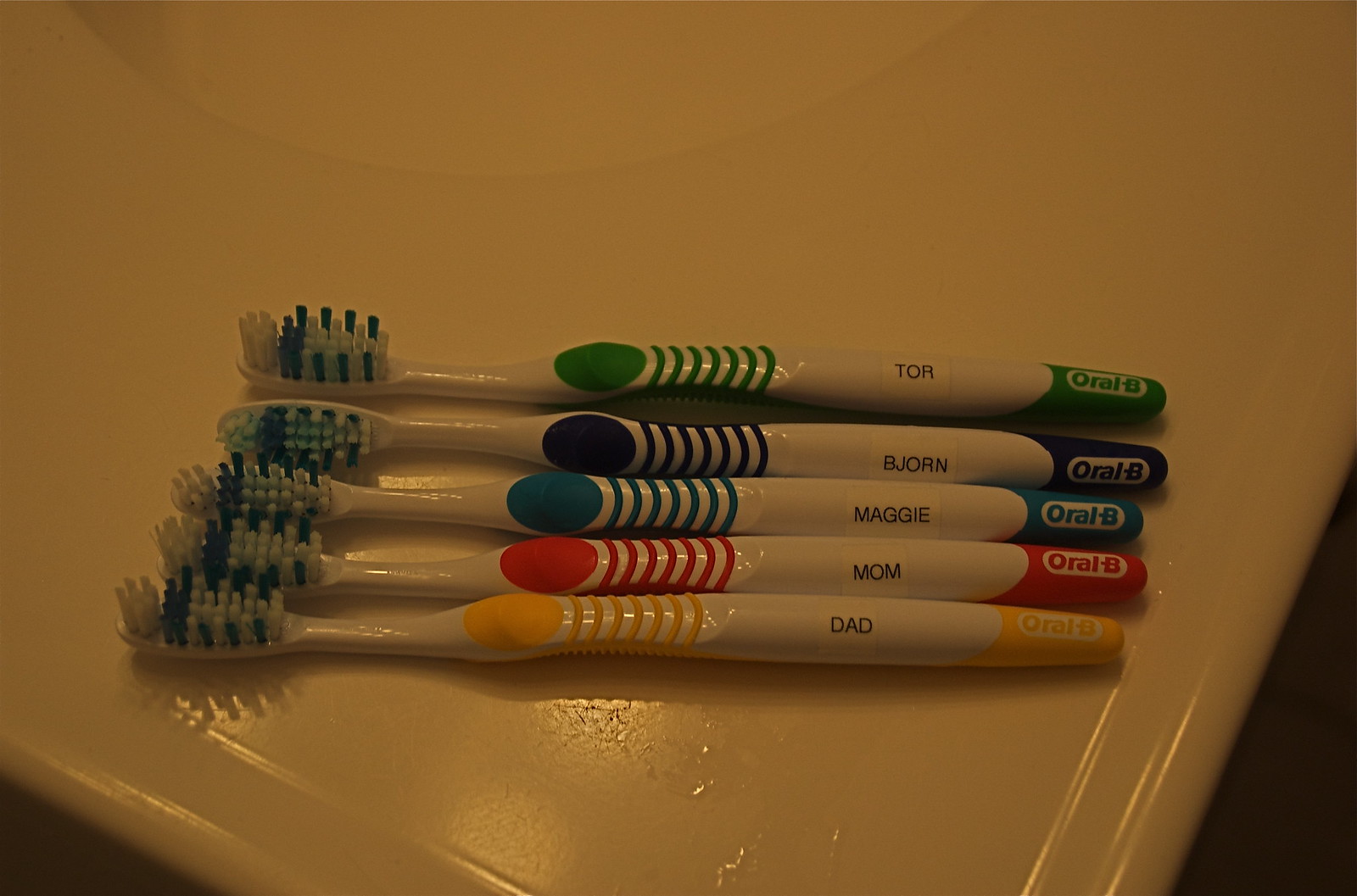This color photograph, rectangular and horizontal in orientation, captures a dimly lit bathroom. Illuminated by a single yellow light bulb, the scene exudes a warm, yet dark ambiance. Central to the image is the edge of a beige bathroom sink, with noticeable water spots and a hint of brown discoloration in the lower right-hand corner.

Arranged neatly on the sink are five Oral-B toothbrushes, each distinctively colored and labeled with names, seemingly belonging to a family. From top to bottom, the green toothbrush is marked "Thor," the dark blue one is "Bjorn," the light blue is "Maggie," the red is "Mom," and the yellow is "Dad." These names hint at a familial structure, possibly with Scandinavian roots. The meticulous arrangement and labeled brushes add a personal touch to the otherwise mundane bathroom setting.